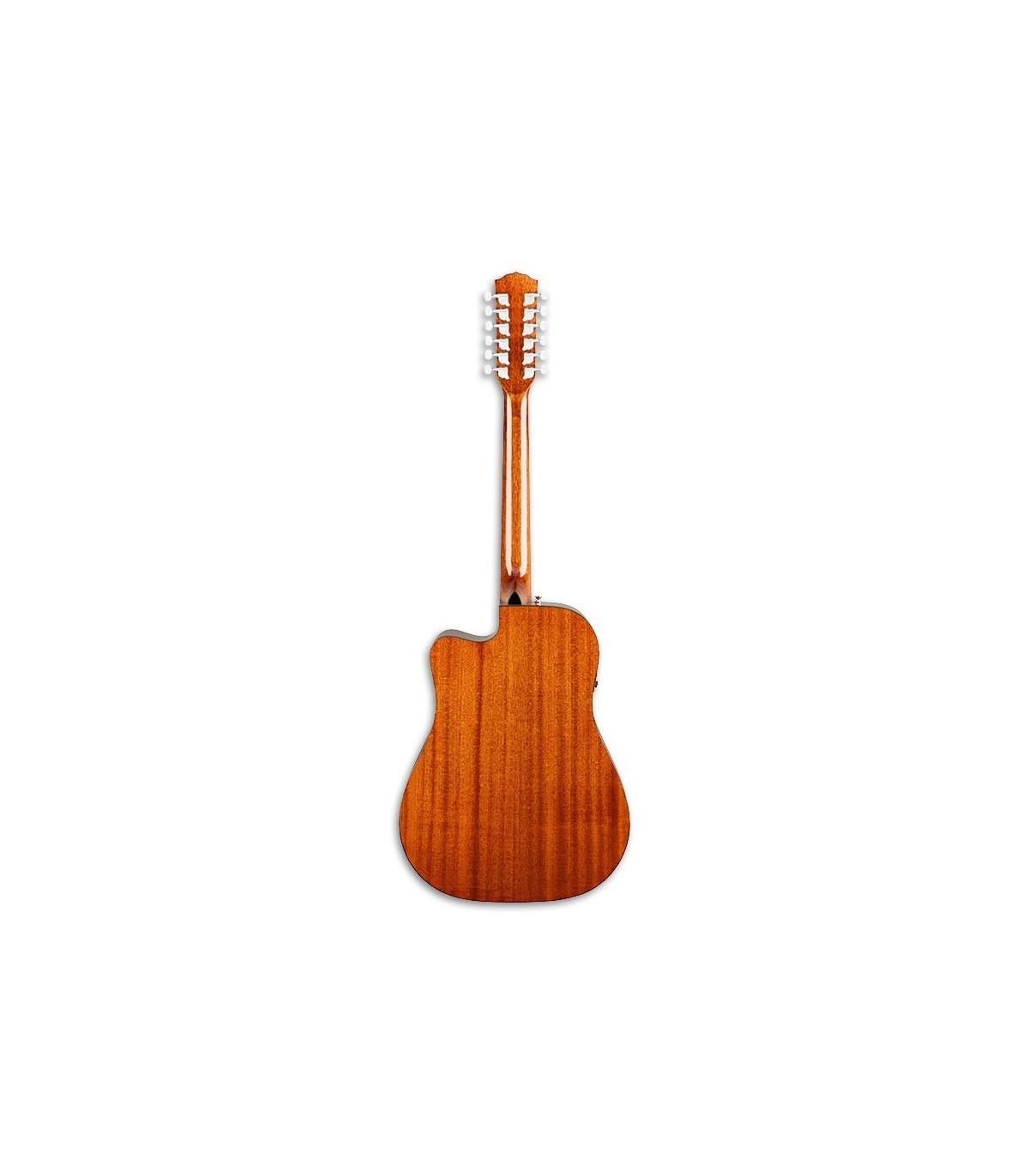The image showcases the back of a guitar, isolated against a white background. The guitar features a traditional body shape and is crafted from a richly colored reddish wood. The hue of the wood darkens slightly towards the bottom of the guitar, creating a subtle gradient effect that is accentuated by natural striped patterns running vertically up the body. The back of the neck continues the reddish wood theme and is adorned with fine white lines along both the left and right edges. These lines highlight the sleek contour of the neck as it extends towards the headstock. The headstock itself is equipped with tuning pegs, adding a practical element to the guitar's elegant design.